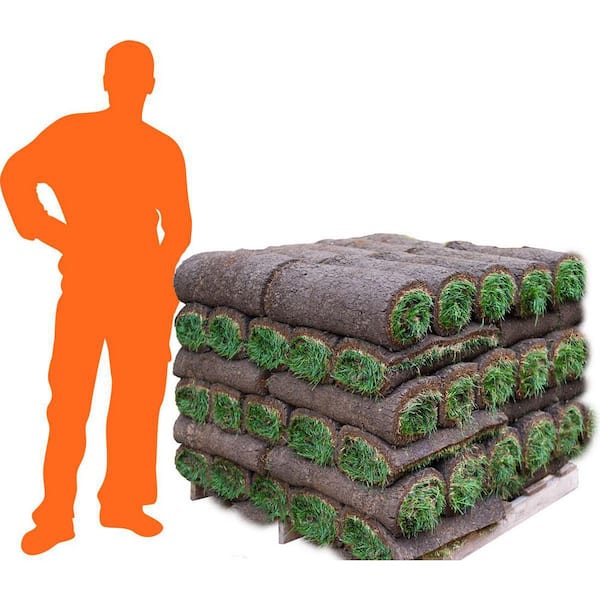In this image, there is a striking silhouette of a man, colored in orange, with his hand on his hip. The silhouette stands to the left of a stacked pile of pre-packaged sod rolls, all positioned on a grey wooden pallet against a white background. The sod rolls, resembling oversized burritos, display a brown, crusty dirt exterior with green grass rolled within. Each roll is neatly stacked in alternating layers, with five rolls per row and a total of six layers, forming a substantial, organized square-shaped pile. The orange shadow next to the sod provides a sense of scale, emphasizing the height and volume of the neatly arranged grass rolls.